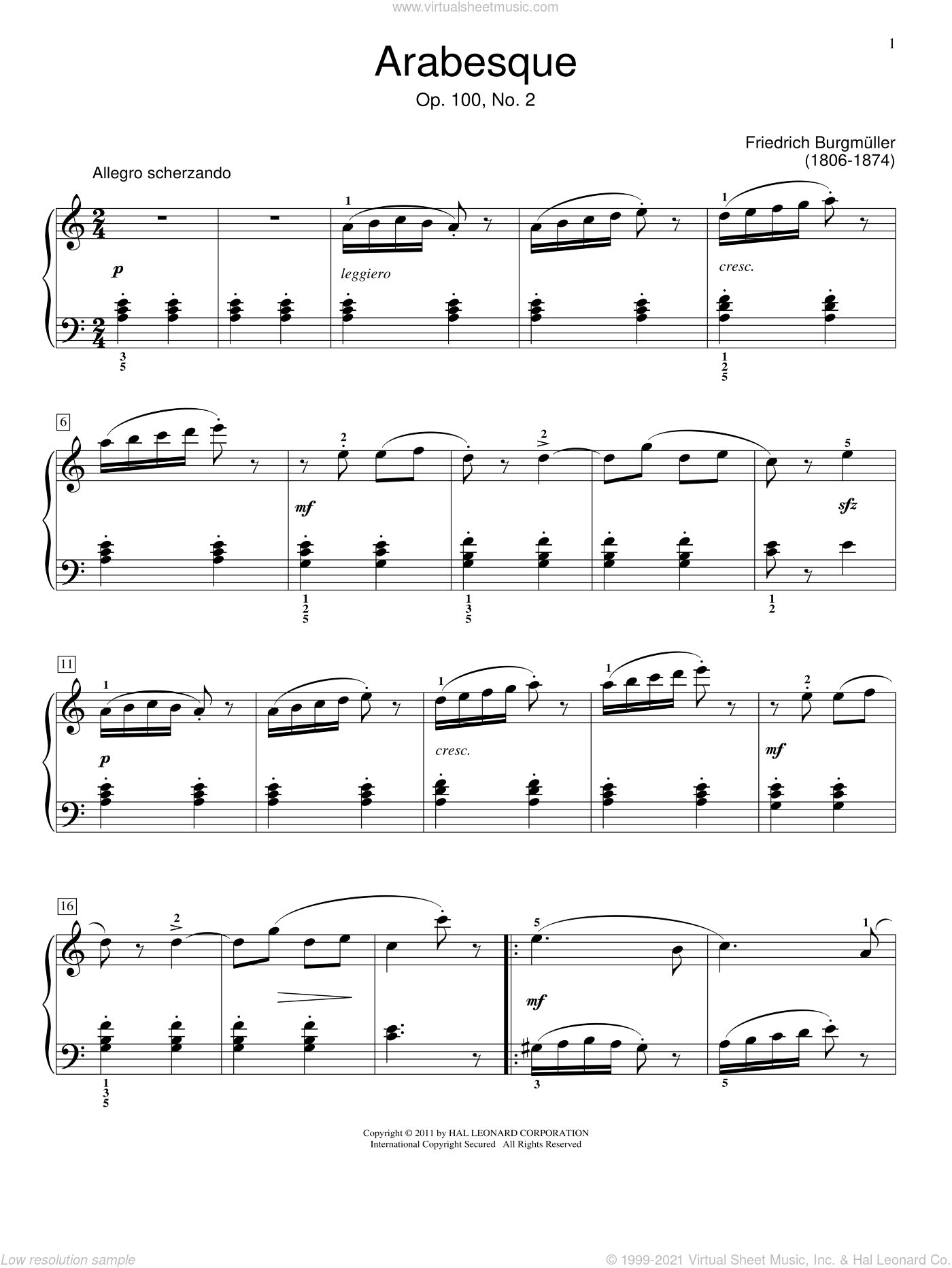This black and white photograph captures a piece of sheet music titled "Arabesque," spelled A-R-A-B-E-S-Q-U-E. The composition is identified as Opus 100, Number 2 by Friedrich Burgmüller, who lived from 1806 to 1874. The sheet features four distinct lines of musical notes, each presenting a different arrangement of the piece. At the top left of the music, the term "Allegro Scherzando" is noted, indicating the tempo and style of the piece. In tiny print at the bottom, it mentions "Copyright 2011 by Hal Leonard Corporation, international copyright secured, all rights reserved." The detailed notation spreads across four rows, offering a comprehensive guide on how to play this specific composition.